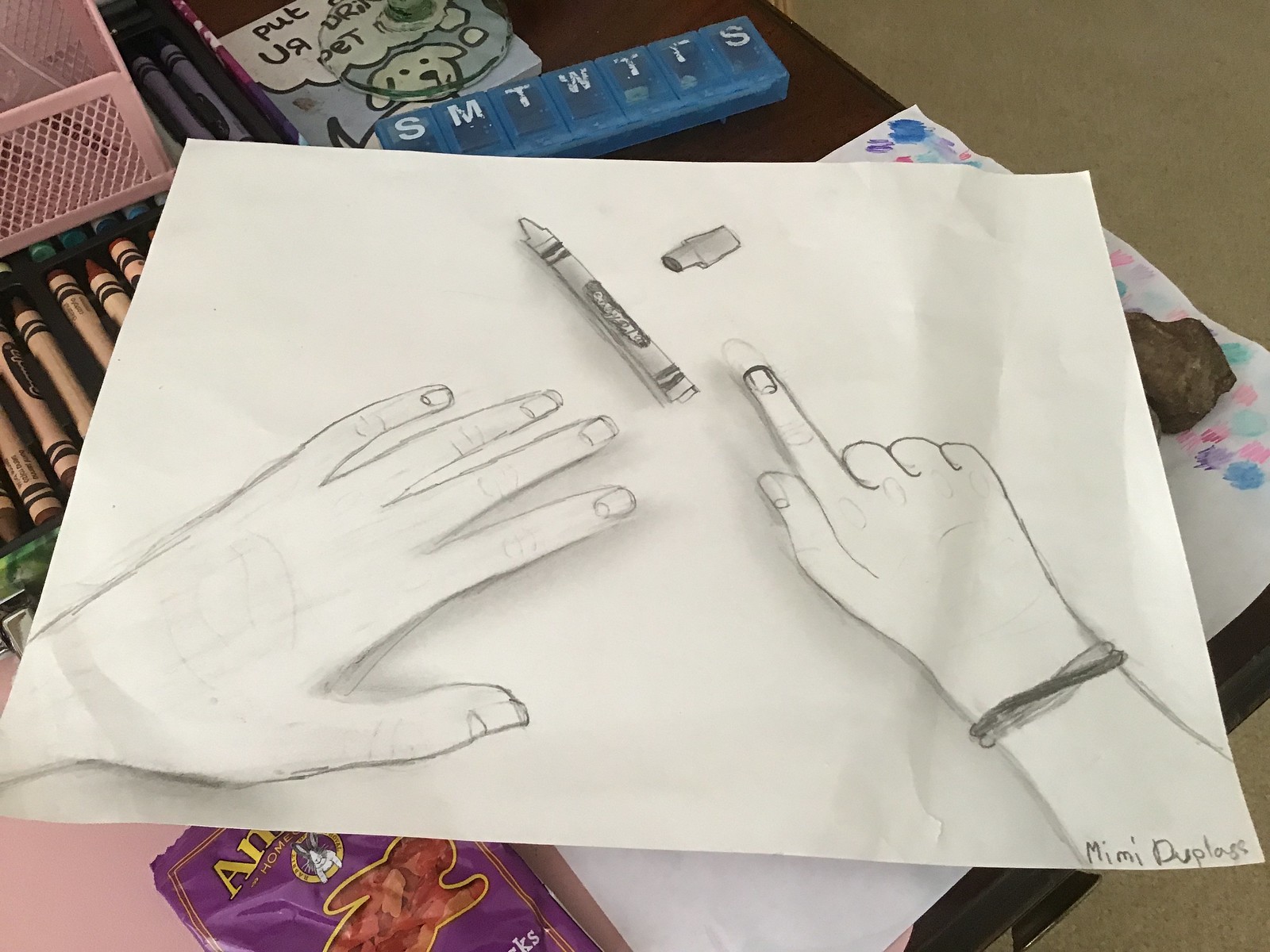The image depicts a vibrant and somewhat cluttered still life scene centered around a childlike crayon drawing. A large sheet of paper, featuring a drawing rendered in pencil or gray crayon, rests on a table. The artwork on the paper illustrates two hands: the left hand is resting palm down, while the right hand is using its index finger to point at a crayon drawn on the paper. 

Surrounding the drawing are various objects, adding context and whimsy to the scene. In the lower left corner, there's a purple packet of what appears to be crackers. To the upper left, an open box of crayons suggests the tools used for the artwork. Centrally positioned at the top of the image, an open book displays a cartoon character of a dog, and nearby sits a small blue box featuring the initials for the days of the week.

The edges of the paper reveal a name written at the bottom left of the sketch, identifying the artist as Mimi Duplass.